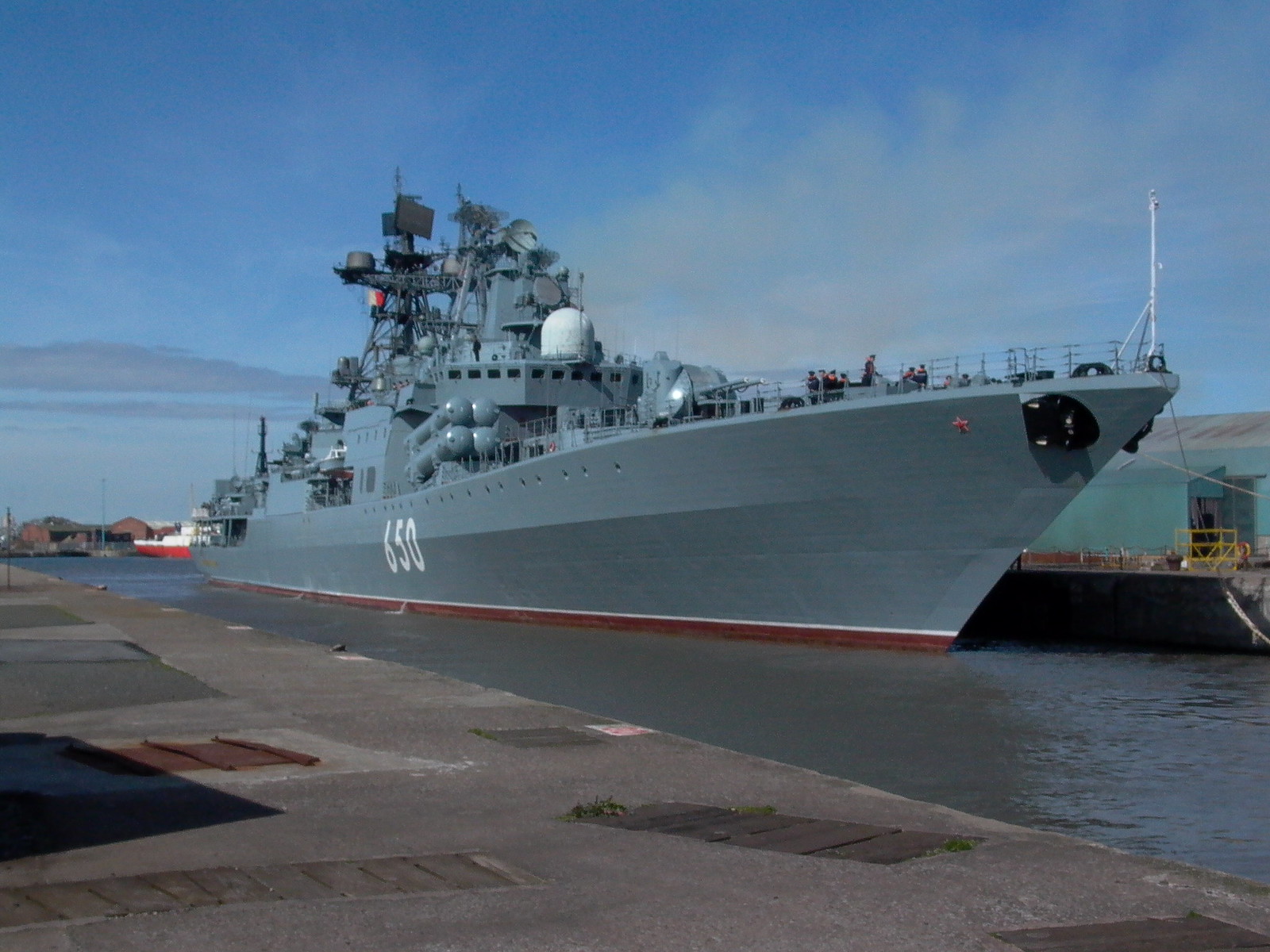The image depicts a teal-colored Navy vessel, numbered 650 in white, anchored on a brownish body of water adjacent to a large cement dock. The ship, with its pointed front facing the camera at an angle, features a maroon line just above the waterline. On the deck, several sailors are gathered near the front, protected by a waist-high wire barrier. A dual-barreled gun turret stands behind them with a reflective white dot. The main part of the ship is populated with an array of equipment including a white dome, numerous satellites, antennas, and what appear to be oil tanks. The bright, sunny day highlights a blue sky dotted with both gray and thin white clouds. In the background, a white and red-bottomed vessel is floating on the water, and the distant shoreline houses some orange-colored buildings with arched roofs.